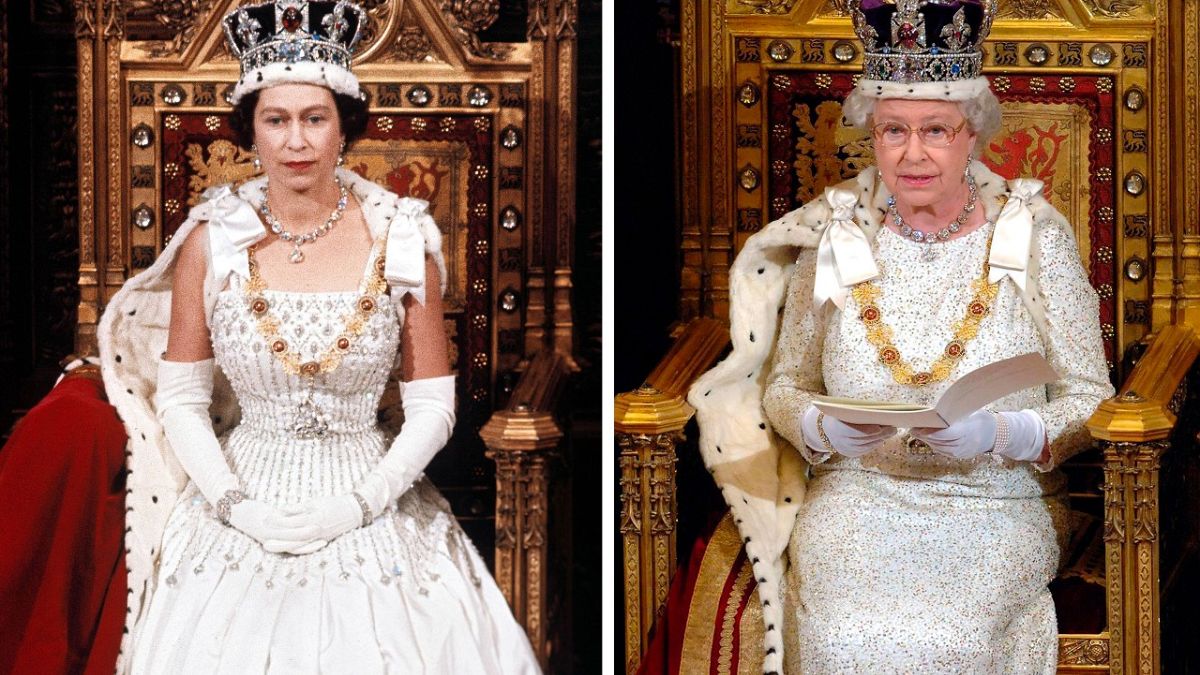The image features side-by-side photos of Queen Elizabeth, highlighting her evolution over the decades. On the left, a young Queen Elizabeth, likely around 26 years old shortly after ascending the throne, sits regally with her arms folded, looking into the distance. She dons a pristine white dress adorned with a gem necklace and earrings, a royal crown atop her black hair, white gloves extending past her elbows, and diamond bracelets on both wrists. A luxuriant thick red royal robe drapes behind her.

On the right, an elderly Queen Elizabeth, appearing in her 80s, is seated on the same throne. She wears a similar white dress with white gloves, a longer necklace, and retains the same regal jewelry, including reading glasses. Her hair is now curly and white, signaling the passage of time. She holds a pamphlet or book in her hands, gazing thoughtfully away from it. Notably, the crown she wears appears slightly larger and higher. Both images capture her enduring grace and regal presence across different stages of her life.